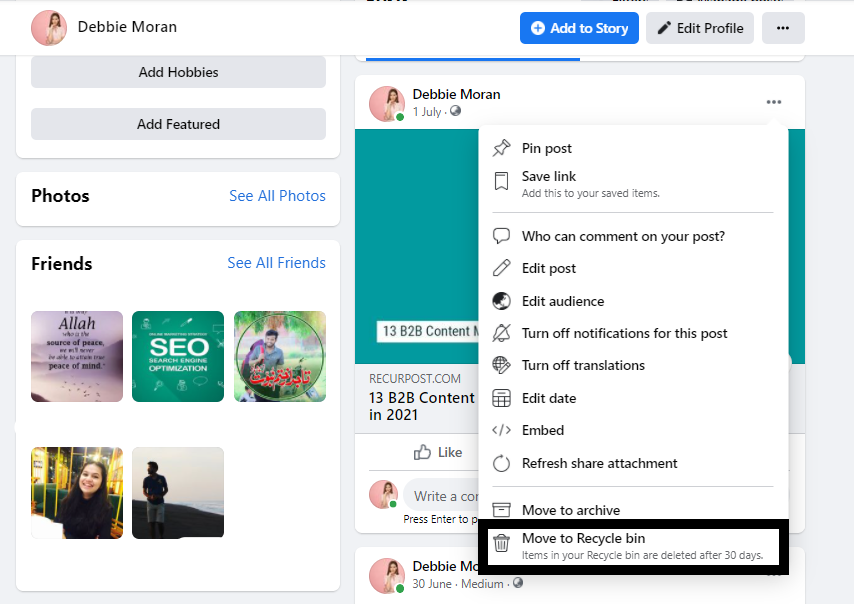This is a detailed screenshot of a Facebook profile page. At the very top, there is a white navigation bar. In the upper left corner, it features the profile picture of a user named Debbie Moran. The profile picture shows a white woman with black hair standing against a beige wall, wearing a white shirt. Next to the picture, her name "Debbie Moran" is displayed in black font.

To the right of her name, there is a blue button with a white plus sign that reads "Add to story" in white font. Adjacent to this button, there is a gray button labeled "Edit profile," which includes an icon of a black pencil.

Below the navigation bar, the screen displays one of Debbie Moran's posts dated 1st of July. She has clicked on her post, revealing a drop-down menu with several options. The drop-down menu has a white background and includes the following options: "Pin post," "Save link," "Who can comment on your post," "Edit post," "Edit audience," "Turn off notifications for this post," "Turn off translations," "Edit date," "Embed," "Refresh," "Share attachment," "Move to archive," and "Move to recycle bin." The "Move to recycle bin" option is notably highlighted with a thick black rectangle, possibly to indicate a focus on how to recycle the post.